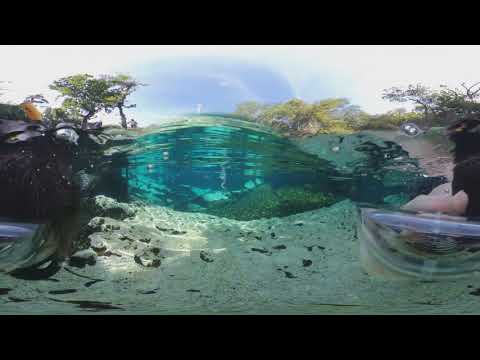In the panoramic photograph of a tranquil lake, the clear, sunlit water reveals a bright blue hue with deeper patches of dark blue, and is dotted with floating algae. The shoreline is sandy with some scattered rocks, casting shadows across parts of the ground while others bask in a lime-green glow under the sunlight. On the right side of the image, there’s a person resting on a transparent purple seat, their legs dipping out of view, possibly into the water. To their side, the sandy ground transitions to a darker, shaded area where algae congregates. On the left, black masses, possibly wet dirt or dense weeds with an orange flower at the top, stand out against the landscape. The image is framed by trees with yellowish-green leaves on both sides. In the background, there’s a clear blue sky with a few white clouds and, intriguingly, what appears to be a lighthouse in the center distance. The serene scene captures the interplay of sunlight and shadow, the reflective quality of the water, and the natural elements surrounding this peaceful waterfront.